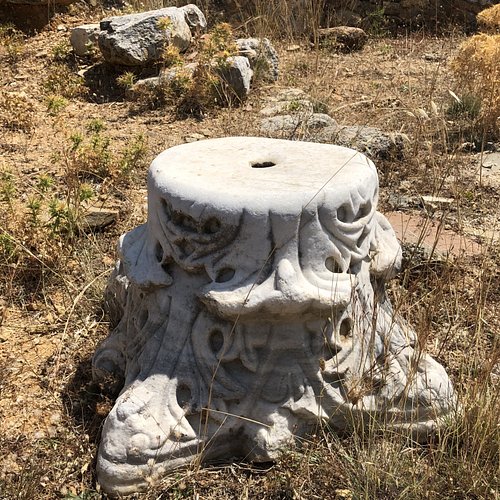In the midst of a dry, rocky, and grassy field, a striking white stone pedestal stands prominently. The pedestal, sculpted with intricate details, features a circular top with a central hole. The structure of the pedestal includes multiple shapes aligned in a pattern that alternates between lines and circles, creating an ornate design. At its base, protrusions resembling feet offer balance and stability. The weathered stone appears to have a whitish-gray hue with hints of yellow and green tints due to age and exposure. Surrounding chunks of tipped-over rocks and dried grasses frame the pedestal.

Closer inspection reveals the pedestal is an artistic statue, creatively carved to resemble a tree trunk with a face. The top features swirls mimicking hair, with broad eyes and a prominent nose positioned beneath. Subtle shadows at the bottom may suggest lips, while holes under the nose add to its mystique. Despite its intricate carvings and dragon-like essence, the statue shows signs of wear, with notches and holes hinting at the passage of time. The pedestal resides amidst scattered dirt, twigs, and the overall arid environment, contributing to its otherworldly and weathered appearance.